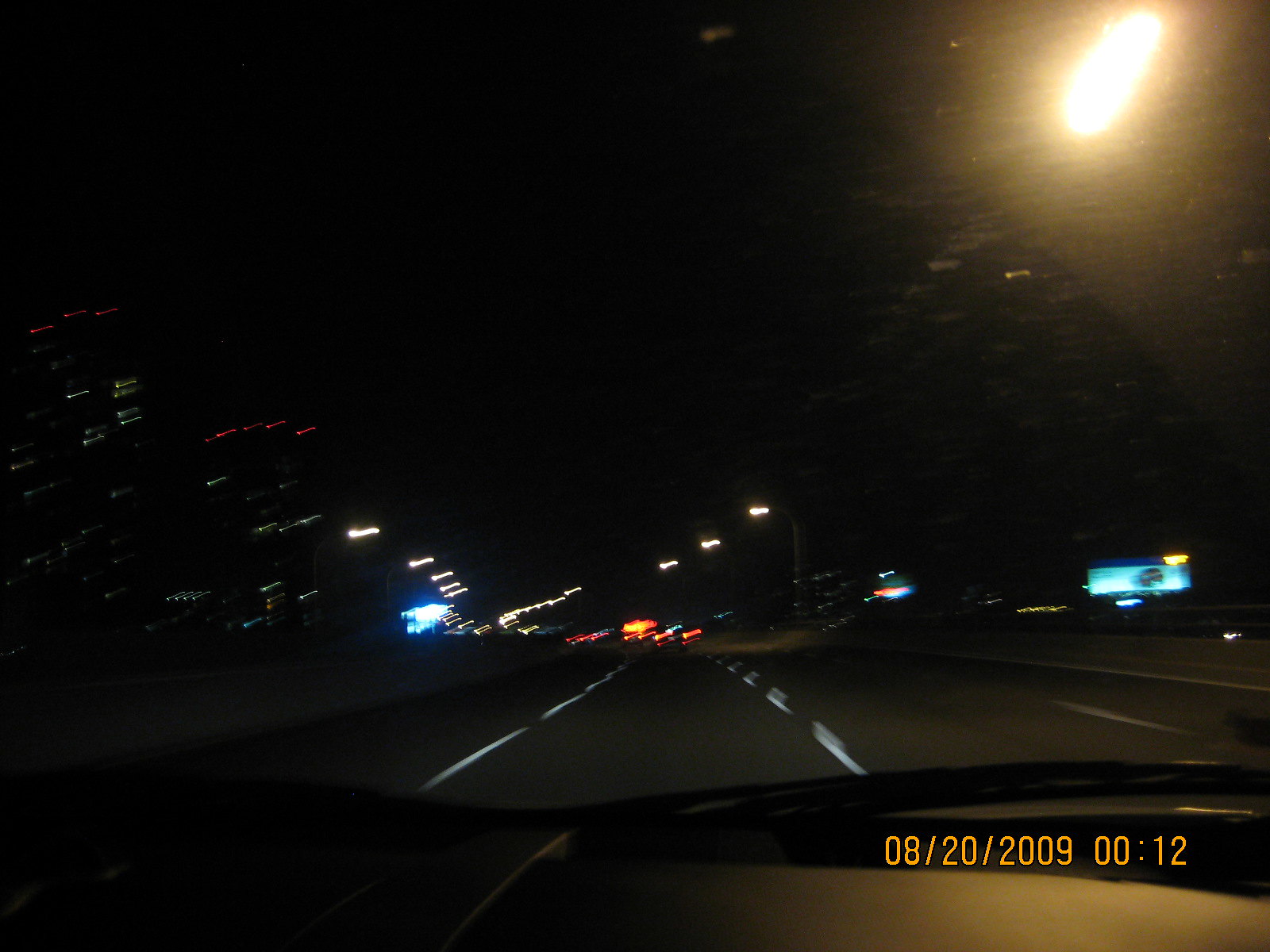This nighttime photograph, taken from inside a car through the windshield, captures the view of a busy highway. The scene is illuminated by numerous streetlights lining the road, casting a warm glow on the vehicles ahead, each with their headlights on. To the left, beyond the cement divider, the skyline is punctuated by tall, illuminated buildings, adding an urban contrast to the scene. On the right, in the distance, a large billboard stands out with its light blue and dark blue hues. The white dashed lines down the middle of the road guide the path forward, adding depth to the composition. The dark sky overhead frames this bustling nocturnal transit scene.